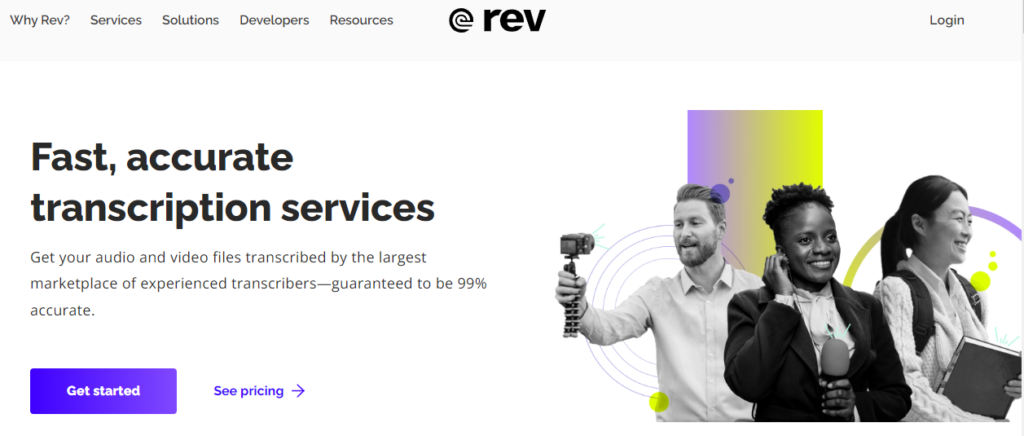The image is a horizontally oriented screenshot of the REV website. At the top center of the image, the word “REV” appears in small, blocky black font accompanied by an address bar. To the left, a vertical menu lists categories titled YREV, Services, Solutions, Developers, and Resources. At the top right corner, there is a “Login” button.

The main section of the image is split into two parts: text on the left and a photographic illustration on the right. The text side prominently features a bold black headline reading “Fast Accurate Transcription Services.” Below this, in smaller text, it explains, "Get your audio and video files transcribed by the largest marketplace of experienced transcribers guaranteed to be 99% accurate." Underneath this description is a purple “Get Started” button. Adjacent to this is another prompt labeled “See Pricing.”

On the right side of the image is an artfully edited black-and-white photograph adorned with purple and yellow illustrated filters. This photograph depicts three people: a man on the left, a woman in the center, and another woman to the right holding a book.